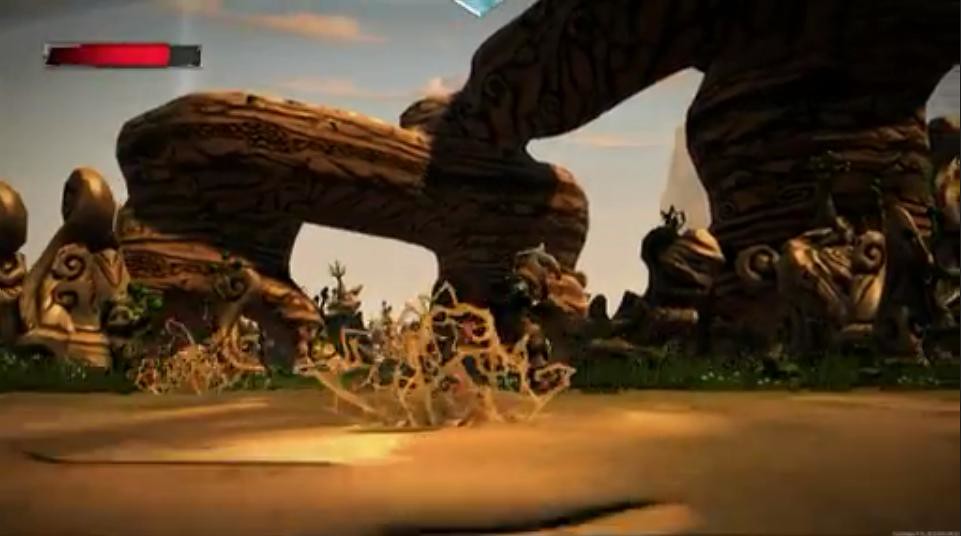In this screenshot from an older video game, the quality is noticeably lower than modern games, with a slightly out-of-focus image. The scene depicts a desert landscape occupying the lower part of the image. The desert floor is dotted with what appears to be white tumbleweeds scattered across it. Prominently in the center of the frame, there are several brown rock formations, one of which arches gracefully from left to right, resembling a natural bridge. To the right of the rock formations, patches of green grass add a burst of color to the otherwise arid setting. The backdrop features a vivid blue sky with scattered white clouds, enhancing the contrast between the earth and the heavens. At the very top of the image is a horizontal health bar: 75% of it is red, indicating the player's health status, while the remaining 25% is black, with a thin white border outlining the bar. Above this bar, some blue text or symbols are present, though they are unclear. Overall, the scene beautifully captures a desolate yet intriguing desert environment from a vintage video game.